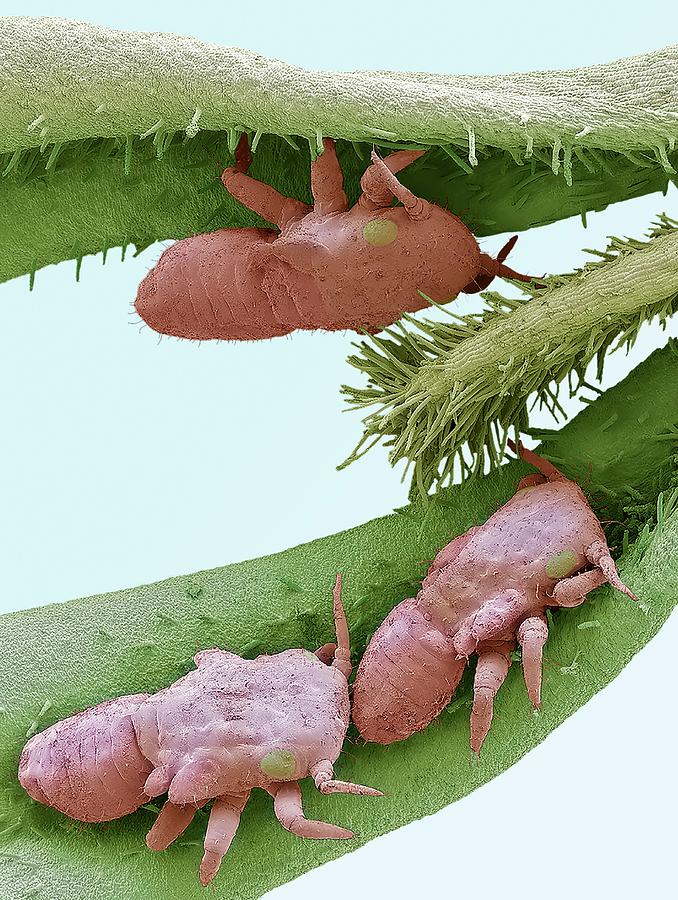This image is a vertically aligned rectangular picture with a light grayish-blue background, featuring a close-up, possibly microscopic or computer-generated view of a plant with green leaves and tiny, detailed spores. The leaves have prickles and sharp tips, with one leaf extending from right to left at the top, a partially grown leaf just below it, and another full leaf stretching downward from the right. Crawling on these leaves are three peculiar, pink-colored critters that resemble wrinkly, potato-like insects or pests. These creatures have little hair-like fuzz and appear to have tails and multiple legs—four on each side. One of these pests is hanging upside down on the topmost leaf, while the other two are on the lower leaves. Despite their detailed features, including tiny hairs and possibly circular yellow eyes, their specific identity remains uncertain.